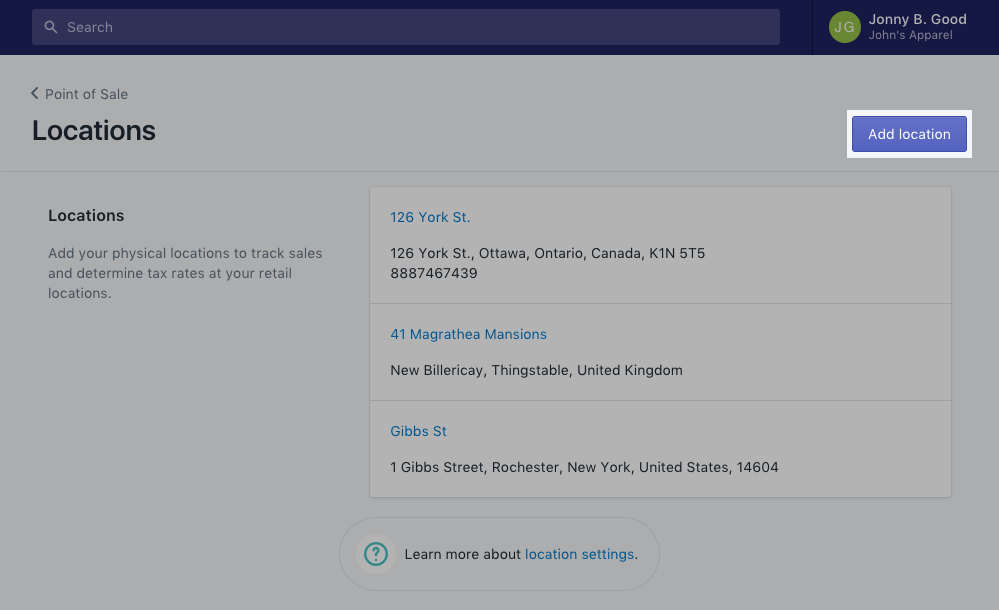The image captures a detailed interface for managing point of sale locations. At the top, there's a search bar prominently displayed. Below that, the title "Johnny B. Good, John's Apparel" is prominently featured, indicating the brand being managed. 

Further down, there's a section prompting users to "Add your physical locations to track sales and determine tax rates at your retail locations." 

Three specific locations are listed:
1. **126 York Street, Ottawa**
2. **41 Magrathia Mansions, New Billeries, Thingstable, United Kingdom (appearing as "Billeries, Billery K" which may denote a formatting issue, spelled B-I-L-L-E-R-I-E-S-Y, Billeri C)**
3. **1 Gibbs Street, Rochester, New York**

At the bottom, there's a prominent button labeled "Add Location" for users to input additional retail locations.